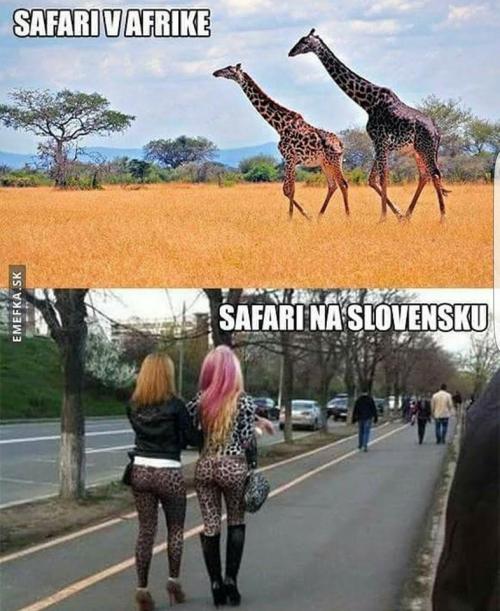A split-image poster contrasts two scenes under identical "Safari" headings. The top half, labeled "Safari V Afrike," depicts two giraffes walking through the arid landscape of what appears to be the Sahara. The field features sunlit, brown and orange grass, flanked by dead trees in the background. The giraffe on the right appears darker and seems sweat-soaked. The sky above is a vivid blue with scattered clouds.

The bottom half, labeled "Safari Na Slovensku," showcases a bustling city walkway lined with trees and bordered by roads. Two women dressed in animal print outfits stride confidently down the path. The woman on the right, with pink and yellow hair, sports a black leather jacket, cheetah-print pants and shirt, and knee-high black boots. Her companion, with short blonde hair, wears animal-print clothing and platform high heels. The street is busy with other pedestrians and traffic against a backdrop of buildings and natural greenery.